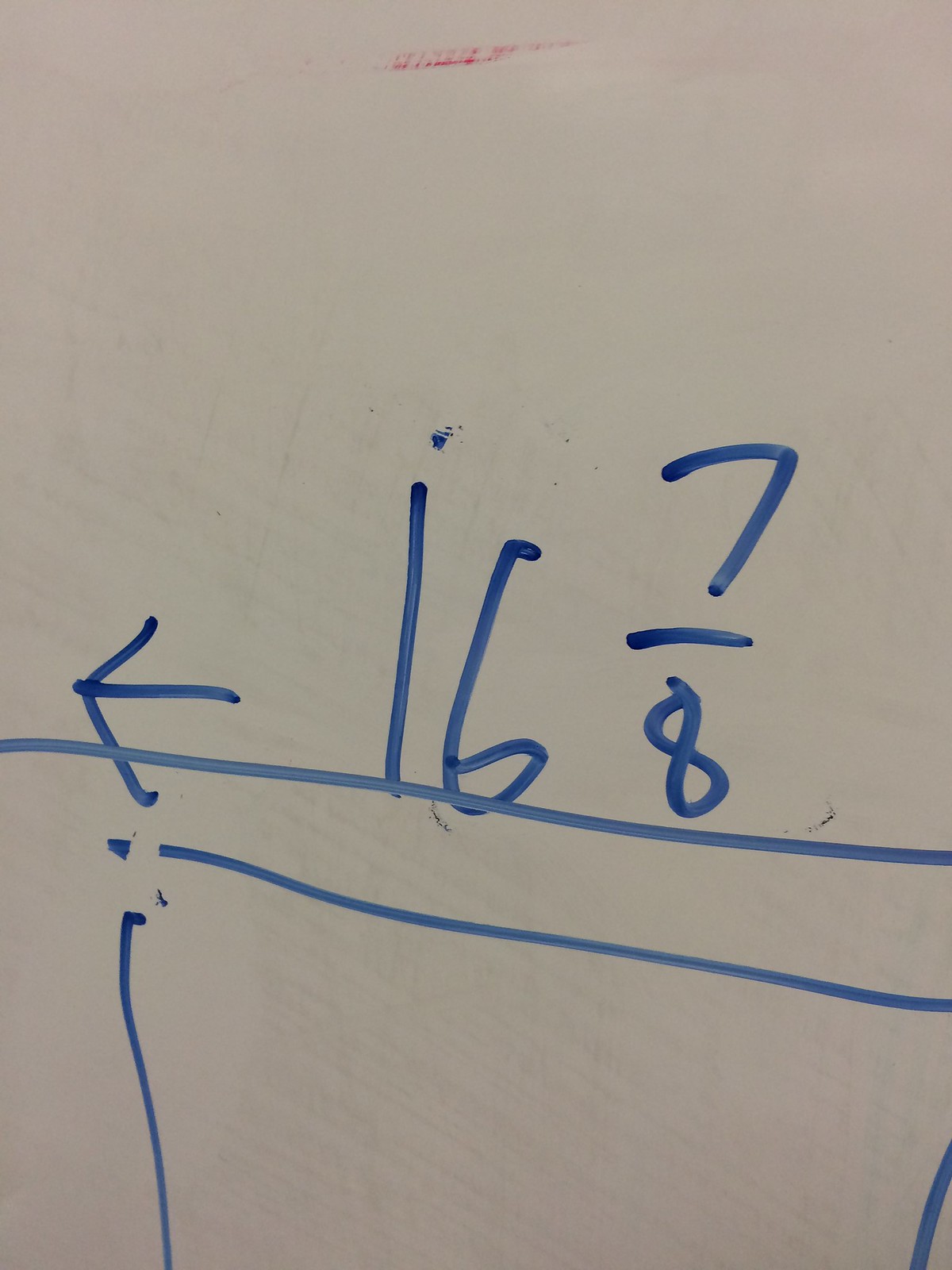The image features a whiteboard primarily filled with a fractional equation written in blue pen. The equation prominently displays the number "16" followed by the fraction "7/8", denoted with the numerator 7, a horizontal dash, and the denominator 8. The whiteboard shows signs of extensive use, with numerous faint markings indicating where previous writings have been erased. This suggests that the board is likely in a classroom or teaching environment. To the left of the numbers, a blue arrow points inward, and beneath the fraction, a horizontal line extends across the width of the whiteboard. There is also an incomplete square on the left side, with only three sides visible: a vertical line, a horizontal line, and another vertical line descending. The focus of the image is clearly on the numerical content, surrounded by minimal additional markings.